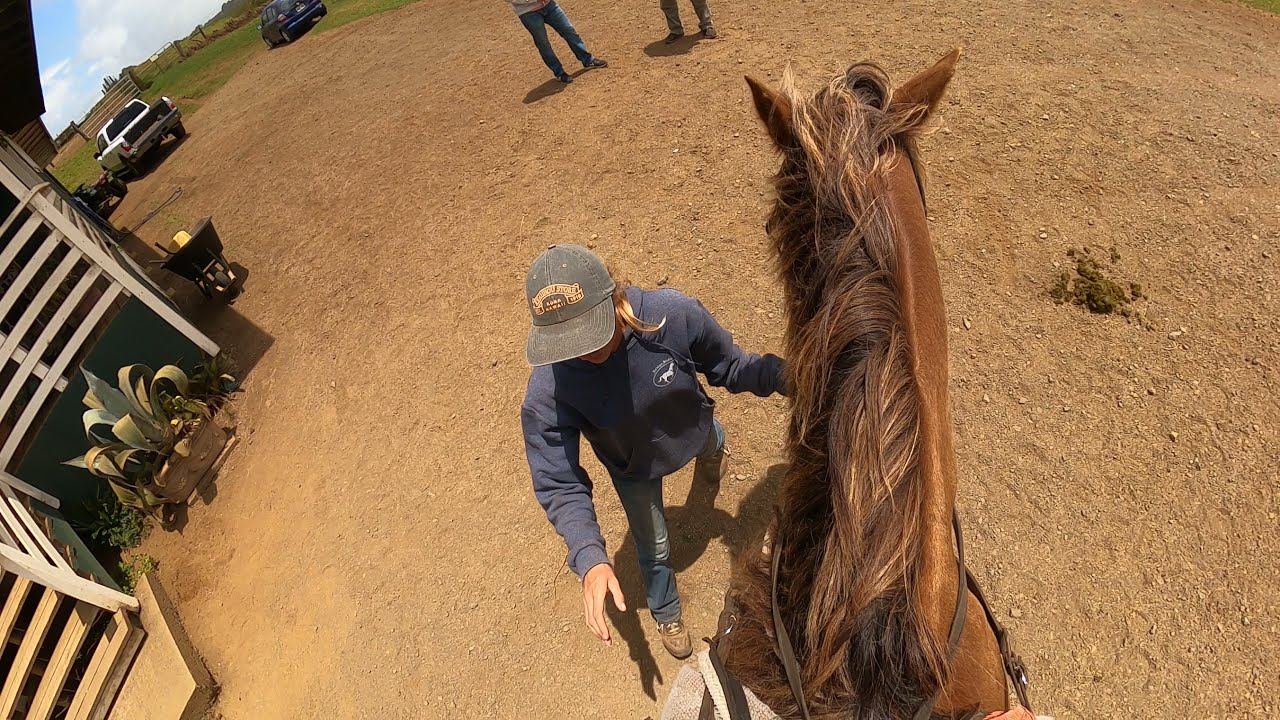From the vantage point of someone sitting atop a brown horse, you can see a detailed outdoor scene on what appears to be a sunny day at a ranch. At the bottom of the image, a hand firmly grips the horse’s reins. Directly ahead, a person with long hair, who looks to be a woman, is wearing a blue shirt, green cap, and blue jeans. She stands facing the horse, either reaching out toward it or the saddle. The dusty, dirt-covered ground stretches across the scene, transitioning into patches of green grass in one corner. To the left of this central action, there's a white-railed staircase attached to a house-like structure. Further details include a couple of vehicles—a white SUV and a blue car—parked nearby. In the distant background, two men are partially visible, only their legs discernible from the angle of the image. The setting is filled with muted tones of browns, tans, and grays, complemented by splashes of green and blue, capturing a typical day on a farm or ranch.